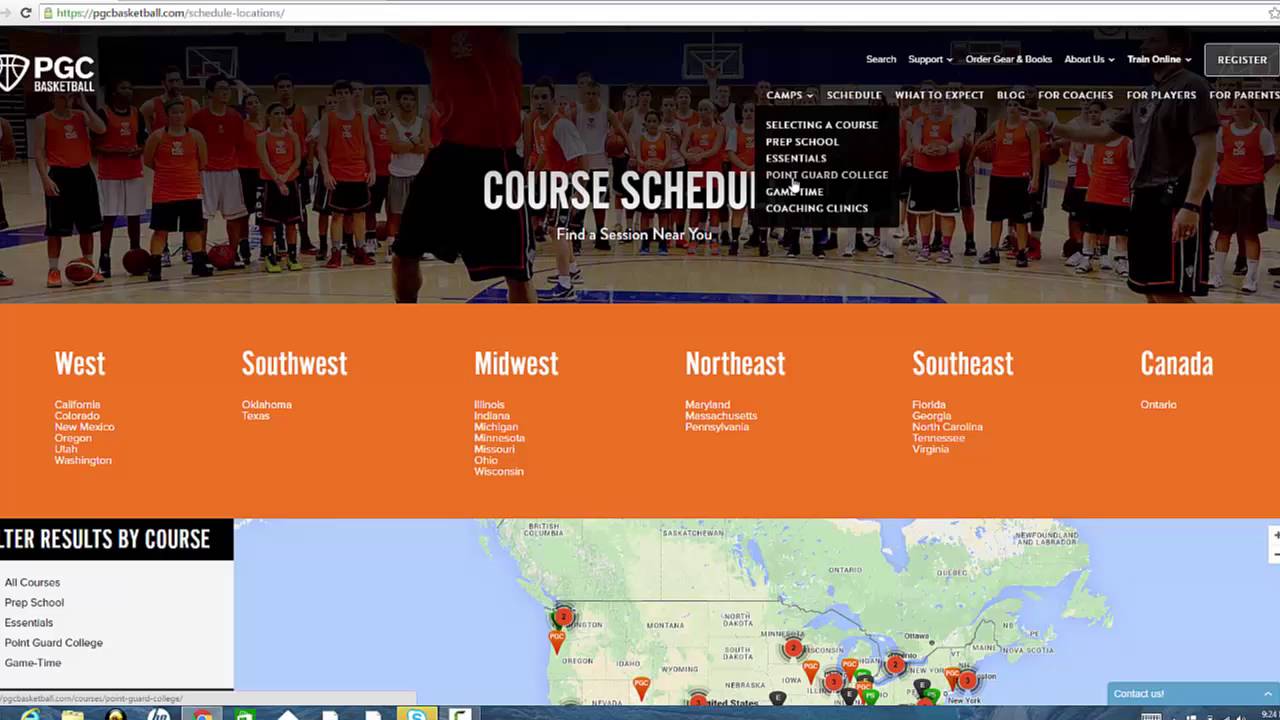The image captures a screenshot of a web page viewed within a browser window, complete with the browser's address bar at the top displaying the URL "pgcbasketball.com". The web page's top third serves as a background consisting of a slightly muted photo of a basketball court, featuring players in red jerseys paired with either black or dark blue shorts. These players appear to be high school-aged.

In the upper left corner of the page, the PGC logo is prominently displayed in large white uppercase letters, with the word "BASKETBALL" in smaller capital letters beneath it. Adjacent to this is an icon resembling a basketball segment shaped like an inverted triangle. 

Centrally located on the page, large white uppercase letters spell out "COURSE SCHEDULE", though the words "L" and "E" are obscured by an active drop-down menu. This menu lists various courses in white font: "Prep School", "Essentials", "Point Guard", "College", "Game Time", and "Coaching Clinics". Adjacent to this, the main menu items are listed from left to right: "What to Expect", "Blog", "For Coaches", "For Players", and "For Partners".

The middle section of the page is characterized by an orange background featuring white text, delineating geographic categories from left to right: "West", "Southwest", "Midwest", "Northeast", "Southeast", and "Canada". Below each heading, the corresponding states where the program is available are listed. Finally, the bottom section of the page displays a partial map, highlighting the northern portion of the United States and parts of Canada with location markers.